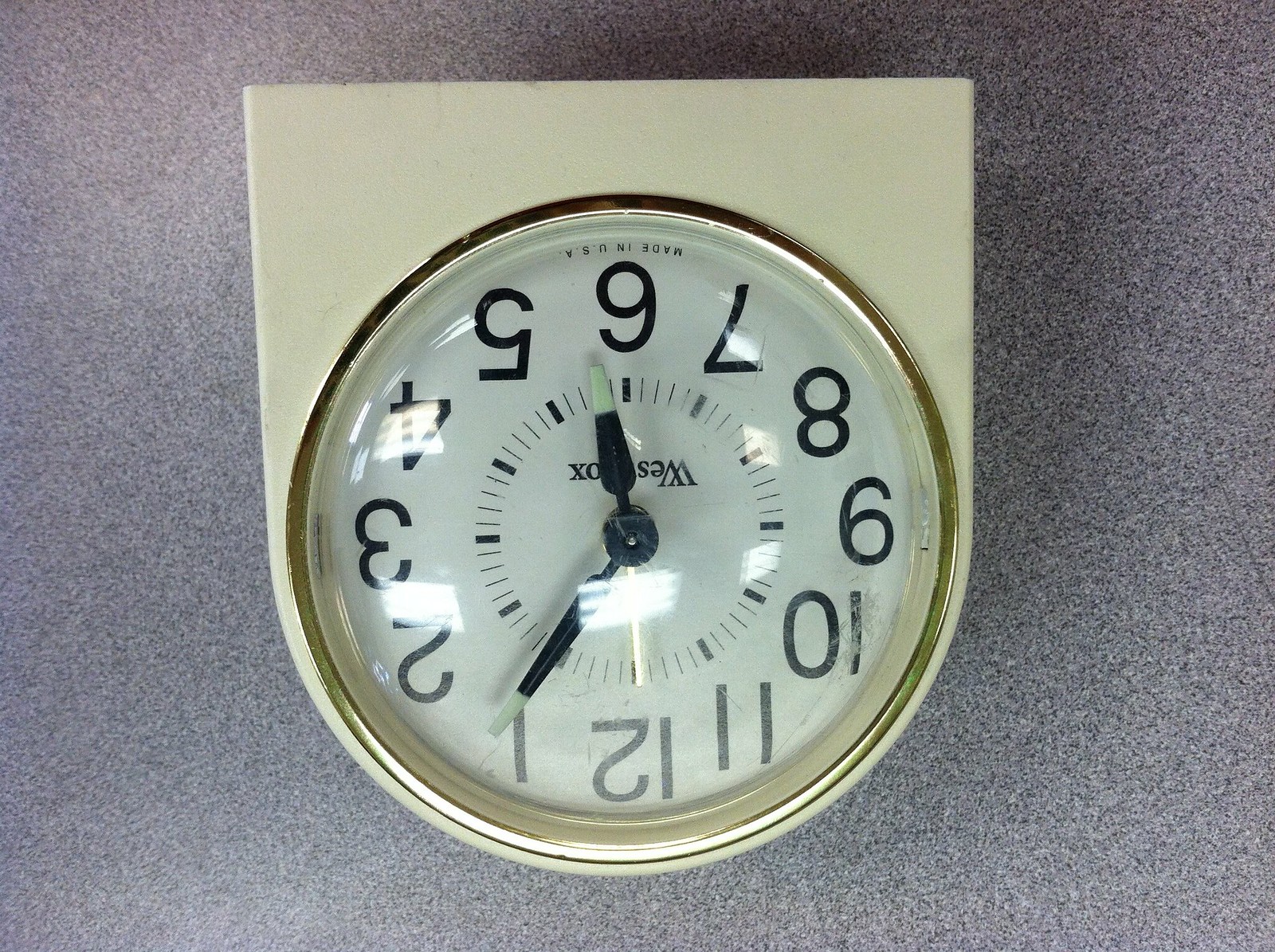In this image, we see a white plastic analog clock that appears to be sitting on a gray, speckled surface, potentially a wall or a counter, though it's unclear. The clock is distinctly upside down with its base at the top of the frame. The clock has a unique design, crafted from cream-colored plastic in the shape of a stacked square and half-circle. It features a round clock face framed by a gold rim and encased in a clear plastic bubble. The black numerals for hours 1 through 12 are visible, though all numbers are upside down due to the clock’s position. The black metal hour and minute hands stand out, both tipped with a glow-in-the-dark green color. The hour hand points near the upside-down six, which now looks like a nine, while the minute hand stretches toward the area where a 1 would be. The brand name "WES-OX" is partly obscured by the hour hand, and “Made in the USA” is printed along the edge under the upside-down 6. This clock is mounted on the surface, adding stability to its displayed position.